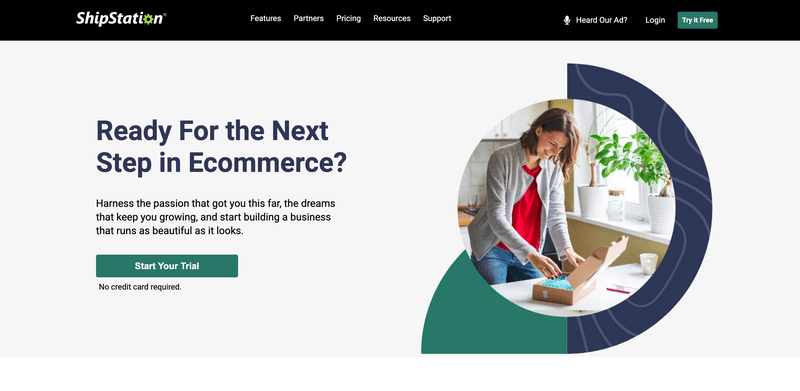In this image from a web page, the design is set against a predominantly white backdrop. At the very top, a black bar spans the width of the page. Within this bar, on the upper left-hand side, the text "SHIP STATION" is displayed in white, with the "O" cleverly replaced by a green gear icon. Moving towards the center, the bar features white text links labeled "FEATURES," "PARTNERS," "PRICING," "RESOURCES," and "SUPPORT" in sequence. Further to the right, there is a white icon resembling a bar, followed by the text "HEARD OUR AD?" and the "LOGIN" button, all in white. The far right of the bar features a green button with the text "TRY IT FREE" in white.

Beneath this black bar, the left-hand side of the page presents an inspirational message in various fonts and colors. In a dark blue font, it states "READY FOR THE NEXT," followed by "STEP IN E-COMMERCE?" directly below. Underneath in black, a motivational phrase reads, "HARNESS THE PASSION THAT GOT YOU THIS FAR, THE DREAMS." Continuing with "THAT KEEP YOU GROWING, AND START BUILDING A BUSINESS." It concludes with "THAT RUNS AS BEAUTIFUL AS IT LOOKS." Below this text, a green bar displays "START YOUR TRIAL" in white, and underneath, in black, it reassuringly states, "NO CREDIT CARD REQUIRED."

On the right-hand side, there is a large circular image featuring a Caucasian woman with shoulder-length brown hair, dressed in a white t-shirt under a gray blazer and blue denim jeans. She is looking down at a white table and is in the process of opening a brown box lined with blue paper. To her right, a windowsill holds two potted plants with vibrant green foliage. The right edge of the circle has a blue border with lighter blue swirling patterns, while the bottom edge has a green-colored border.